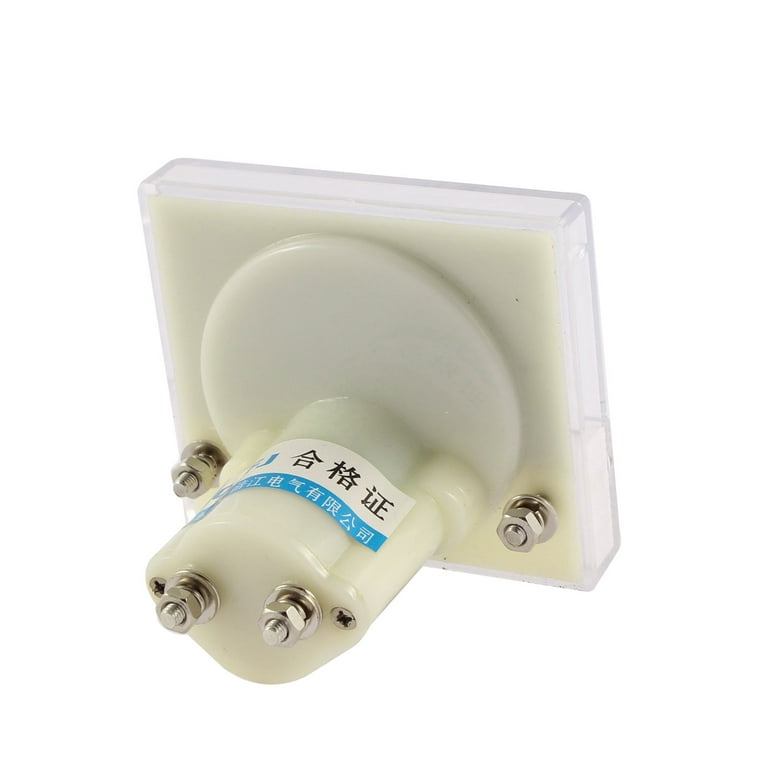This is a detailed color product shot featuring a white, opaque plastic device set against a white background. The device includes a square, clear plastic perimeter at the top and an off-white plastic square section with a circular indentation centered within it. From this circular section, three cylinders extend outward toward the camera, with the central cylinder being thicker than the two on the sides. The contraption is equipped with multiple fasteners: there are four prominent bolts with nuts located at the bottom left and right of the square section as well as on the bottom of the protruding cylinders, all silver in color. Additionally, there are two smaller screws. On the front of the device, near the circular section, there’s a label featuring black Chinese characters against a white background, accompanied by a blue strip with additional white Chinese characters.